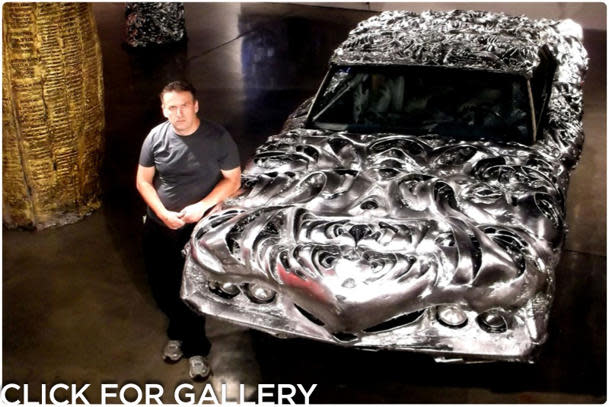The photograph, taken from an overhead perspective, showcases a striking and unusual custom car parked indoors, likely in an art gallery due to the presence of sculptural elements on the left side of the image. The car's exterior is adorned with intricate, sculptural metal ridges arranged in concentric forms, giving it a unique, almost swirly silver texture reminiscent of cake frosting. Leaning on the left side of this futuristic vehicle is a man with short brown hair, dressed in a dark gray shirt, black pants, and gray sneakers. He gazes up at the camera with a serious expression. Additionally, at the bottom of the photograph, there's a white text caption in large, all-capital letters that reads, "CLICK FOR GALLERY," suggesting the image might be from an online exhibit or a website. The polished concrete floor enhances the artistic ambiance of the setting, complemented by the partial view of gold, striated sculptures nearby.